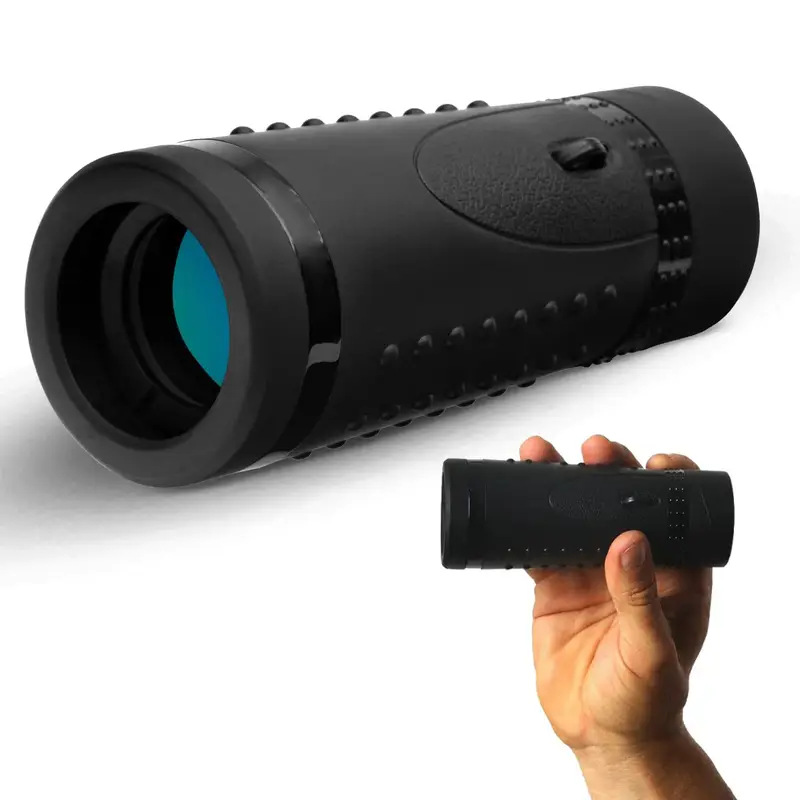This image, which resembles a product advertisement display, showcases a cylindrical black device, likely a monocular viewer or some type of scope. The device is prominently featured at the top of the image, lying horizontally and displayed in high detail against a blank white background. The scope, approximately five inches long, boasts a sleek black design with a blue, translucent lens visible at the open end, hinting at its optical function. The cylindrical body includes several black rivets and textured grip areas for better handling. Some black rings accentuate the edges, enhancing its sleek appearance. Below this detailed shot, a second image depicts a person's light-colored hand holding the scope as one would hold a telescope, though their face is not shown. The hand's positioning, with three visible fingers and a thumb grasping the device, illustrates the scope's compact size and ergonomic grip. The clean, white background and the high-resolution detail suggest that the image is intended for a catalog or online product display, emphasizing the scope's design and functionality.